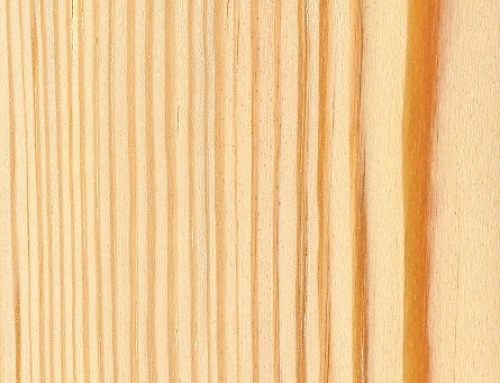This image is a highly detailed macro photograph featuring a close-up view of a wooden surface. The surface, potentially plywood, fills the entire frame, presenting a symmetrical and centralized composition. Vertically running lines are clearly visible, showcasing the grain structure in varying shades of brown and tan, interspersed with darker, almost caramel-colored lines. No text is present, maintaining the natural look of the wood. The intricate layering and vertical alignment might suggest a setting related to construction or a home improvement store, though the specific context remains uncertain. The image's detailed focus on the wood's texture and grain highlights the material's natural beauty.